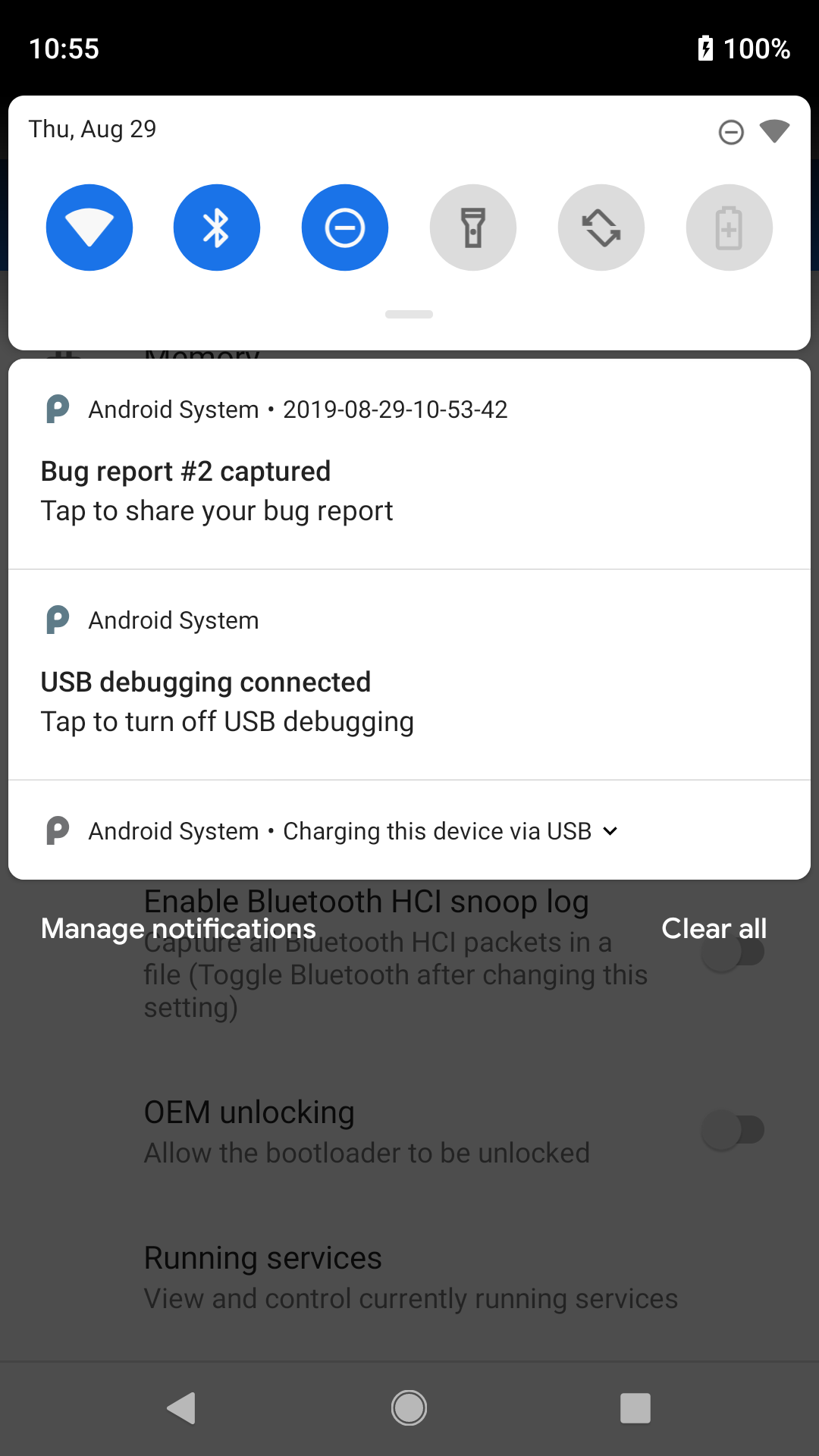In this detailed image of an Android phone screen, situated at the top right corner is the battery icon, which shows that the device is fully charged at 100%. This icon also features a black thunderbolt, indicating that the phone is currently charging. On the top left, the time is displayed as 10:55.

Directly below the time, a white rectangular notification bar spans the screen. At the top left corner of this bar, the date is shown as "Thursday, August 29th." Within this notification bar, there are six distinct circular icons. The first three icons, set on a blue background, represent Wi-Fi connectivity, Bluetooth functionality, and a "Do Not Disturb" mode (a circle with a dash). The next three icons on a gray background indicate a flashlight, a screen rotation lock, and another battery symbol.

Further down, the phone displays several notifications and system messages in separate boxes. These notifications include "Android system bug report number two captured," "USB debugging connected," and "Charging this device via USB." 

In the lower half of the image, additional system options and notifications are visible. They feature options such as "Manage notifications," "Clear all," "Enable Bluetooth ACI," "OEM unlocking," and "Running services." This comprehensive display offers a glance into both the device’s status and ongoing activities.